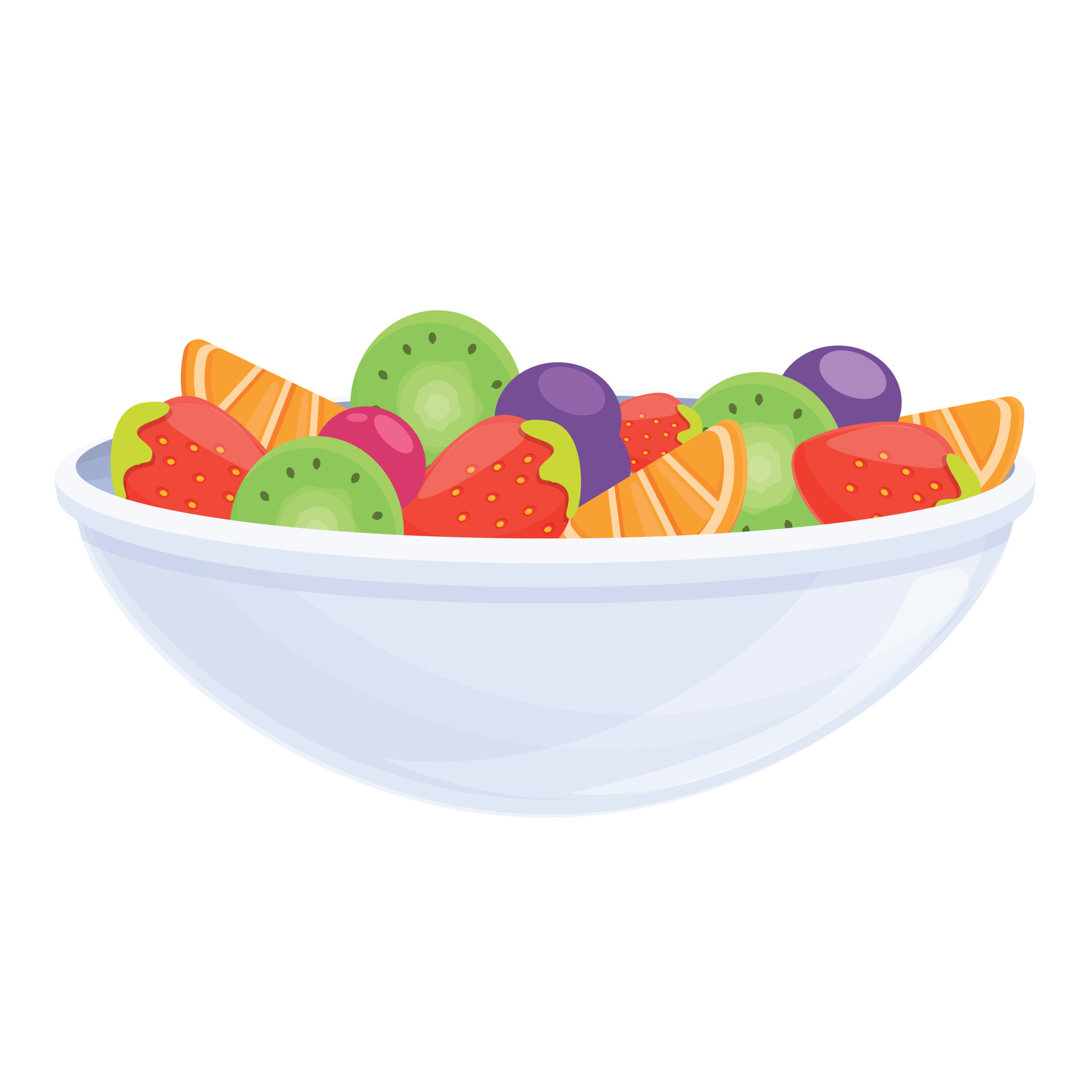This image is a detailed clip art style illustration of a bowl of fruit, floating against a pure white background. The bowl itself is wide and white, with shading that transitions from medium blue-gray to lighter gray, and features a clean white rim. Inside the bowl, there are approximately 14 pieces of various fruits, arranged to resemble a fruit salad. The fruits include light orange slices, whole red strawberries with yellow spots and green leaves, circular slices of light green kiwi with black seeds and pale centers, and two large round purple grapes. Additionally, there is one pinkish-red cherry, which is the same size and shape as the grapes but distinct in color. The intricate details and colors of each fruit are clearly illustrated, making the image vibrant and visually appealing.